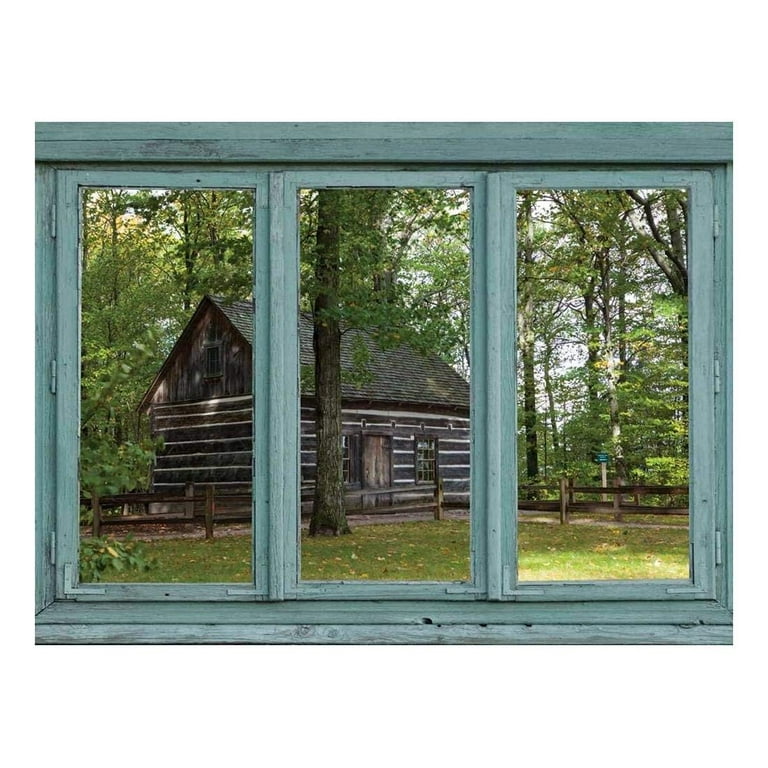Through the large, three-paned window, which is painted a light country blue, we get a clear, un-obstructed view of a rustic scene. This wooden window, devoid of curtains or blinds, frames a weathered log cabin, constructed from dark brown wood, suggesting a seasoned yet recent build. The cabin, which has a typical shingled roof, sits amid a lush, forested area dense with vibrant green trees and foliage. Surrounding the cabin is a quaint wooden fence with a small walkway leading up to it. The scene evokes a serene, country atmosphere, which could likely be a historical site, a cozy lodge, or a retreat, offering a picturesque and tranquil escape into nature.